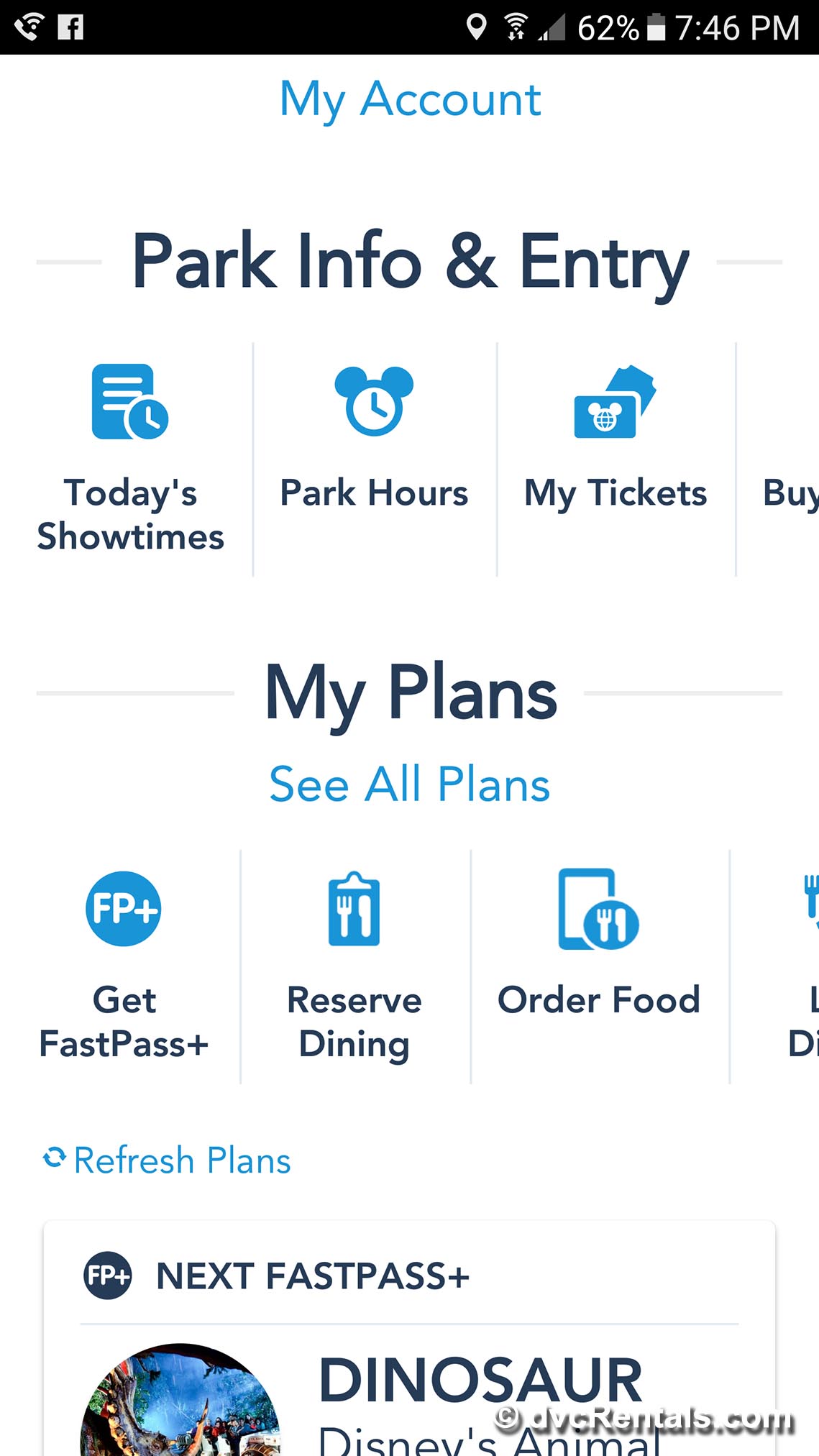The image is a screenshot from a cell phone, likely displaying an app interface. At the very top is a black banner featuring various status icons, including a phone and WiFi signal indicators. There's also a small, white square with a black "F" inside of it. On the opposite side of the banner, it shows the location, WiFi strength, cell signal strength, the battery level at 62%, and the time, which is 7:46 PM.

Below this, the background transitions to white. At the top of this section, in blue font, it says "My Account," with "M" and "A" capitalized. Further down, it displays "Park, Invo & Entry," with "P," "I," and "E" capitalized and an ampersand between the words. Below this, there are several icons labeled "Today's Showtimes," "Park Hours," and "My Tickets."

The next section is titled "My Plans," with both "M" and "P" capitalized. Underneath, there is blue text that says "See All Plans." More icons are below, labeled "Get FastPass Plus," "Reserve Dining," and "Order Food." There is also an option in blue text labeled "Refresh Plans." The final visible section shows "Next FastPass Plus" followed by "Dinosaur Disney's Animal," although the text is cut off, suggesting there is more information not fully visible in the screenshot.